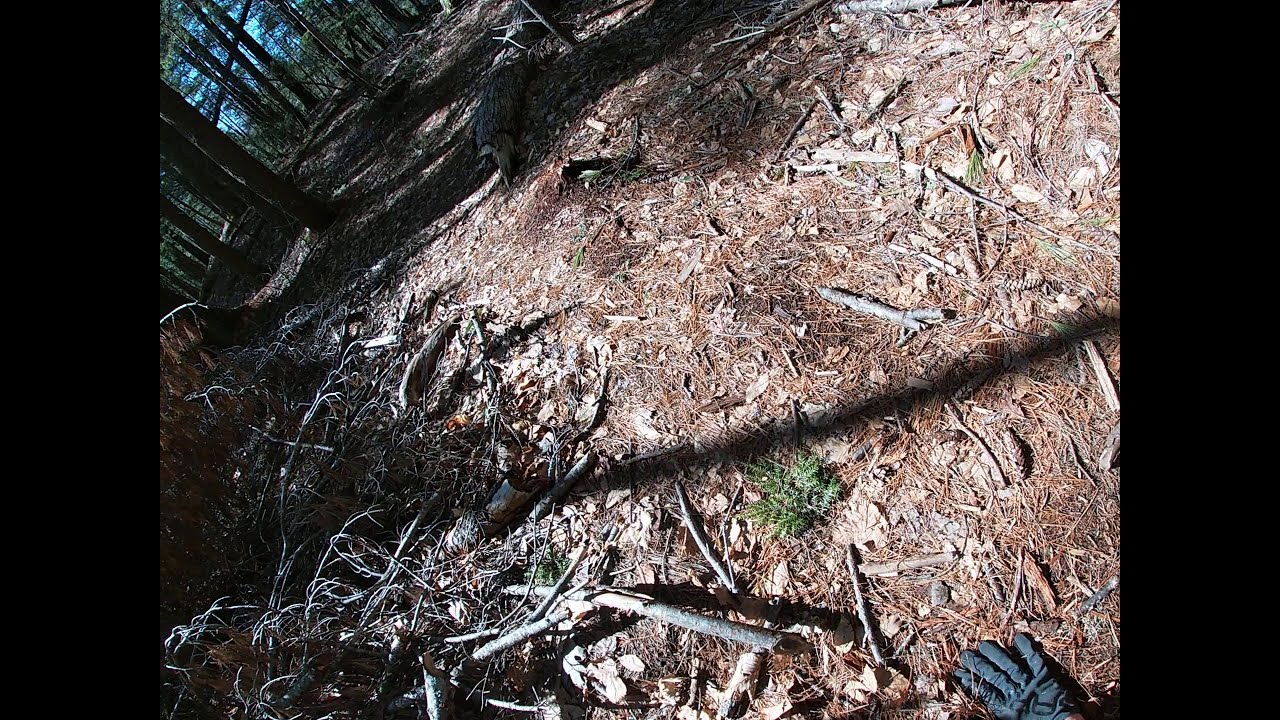In this outdoor daytime photograph, framed vertically with black borders on each side, we observe the forest floor of a wooded pathway strewn with dead sticks, small branches, pine needles, cones, and leaves from both coniferous and deciduous trees. The path runs diagonally from the lower right to the upper left, partially covered with light gray glove-clad hand in the lower right corner, suggesting that the photographer may have fallen and is bracing themselves. The trail meanders through tall, thin trees, with bright sunlight filtering through the canopy, illuminating patches of grass here and there, while a blue sky peeks through the tree line in the background, adding contrast to the natural scene.